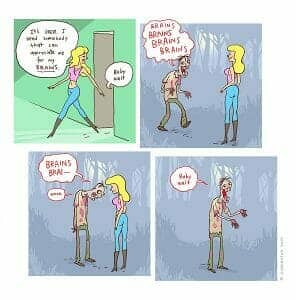The image is a comic strip composed of four panels arranged in a two-by-two grid. The artwork has a pixelated, hand-drawn style reminiscent of comic book illustrations. 

In the top-left panel, a blonde woman with tall boots, blue jeans, and a pink shirt steps out of a door into a green room. She has a speech bubble saying, "I wish somebody would appreciate me for my brains." In the same panel, a voice from inside the room calls out, "Baby, wait."

Moving to the top-right panel, the woman is now standing outside in a gray forest. A zombie approaches her from the left, repeatedly saying, "Brains, brains, brains, brains," in a speech bubble.

The bottom-left panel shifts to a close-up where the zombie, appearing dejected with its head down, continues murmuring, "Brains, brains." The woman looks at the zombie silently.

In the final bottom-right panel, the zombie stands in the middle, still looking disheveled and bloody, with a speech bubble that reads, "Baby, wait."

The storytelling in this comic strip humorously juxtaposes the woman's initial desire to be valued for her intellect with the zombies' literal craving for brains.